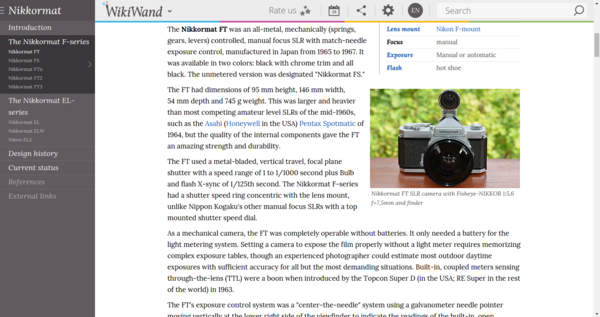The screenshot in question features a wiki-style page, although it is not from Wikipedia. The page seems to be related to a particular camera model, with a layout divided into two main sections. 

On the left-hand side, a gray column contains a navigation menu with the header "NIKKORMAT." The first option listed is "Introduction," followed by other options such as "Design History," "Current Status," "References," and "External Links." The text beneath this column appears to be in low resolution.

Dominating the right-hand side, the prominent header "WIKIWAND" introduces the main content, which provides a detailed description of the NIKKORMAT-FT camera. The NIKKORMAT-FT is described as an all-metal, mechanically controlled manual focus SLR (Single-Lens Reflex) camera with needle exposure control, manufactured in Japan. Its production dates are approximately from 1965 to 1967. The camera was available in two color schemes: black with chrome trim and an all-black version.

Further down the page, an extensive text elaborates on the usage of the NIKKORMAT-FT, which likely includes instructions and specifications. Accompanying the text, there is a small image of the camera. The image depicts an old-style SLR camera with a distinct round protruding element at the top, which could possibly be part of the NIKKORMAT-FT’s mechanism or design features.